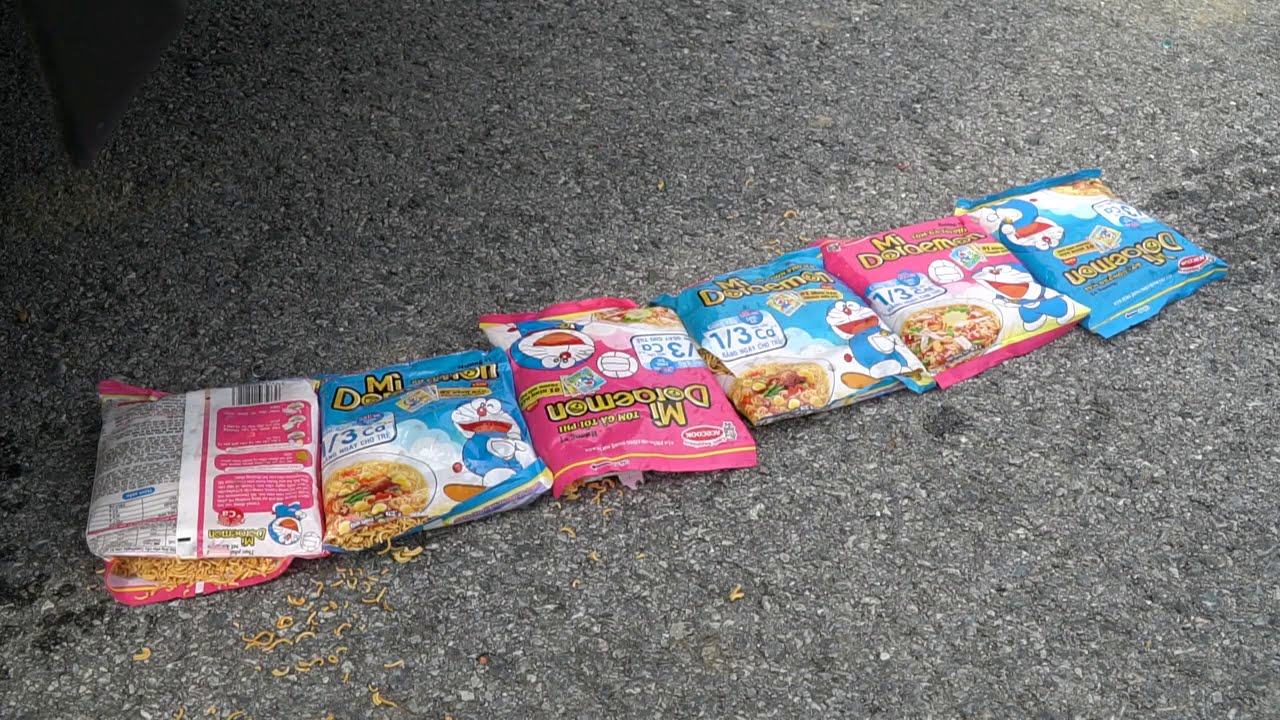This image depicts six packets of instant noodles labeled as "mi dorumian," laid out on a gray, pebbly asphalt surface. The packets alternate between pink and blue colors, arranged in a single row but in varying orientations—some right side up, others upside down, and at least one lying on its back. The mostly blue and pink packages show signs of wear, with crumpled portions and some even appearing to be run over, as indicated by visible tire tracks. One packet on the left is open, spilling some of its dried noodle contents onto the pavement. Each packet features a stylized, somewhat illegible logo and an image of a bowl of noodles along with other graphic elements, contributing to the overall cluttered appearance. The image has a generally dark tone with no clear, bright lighting source, capturing a scene of disarray and rough texture.